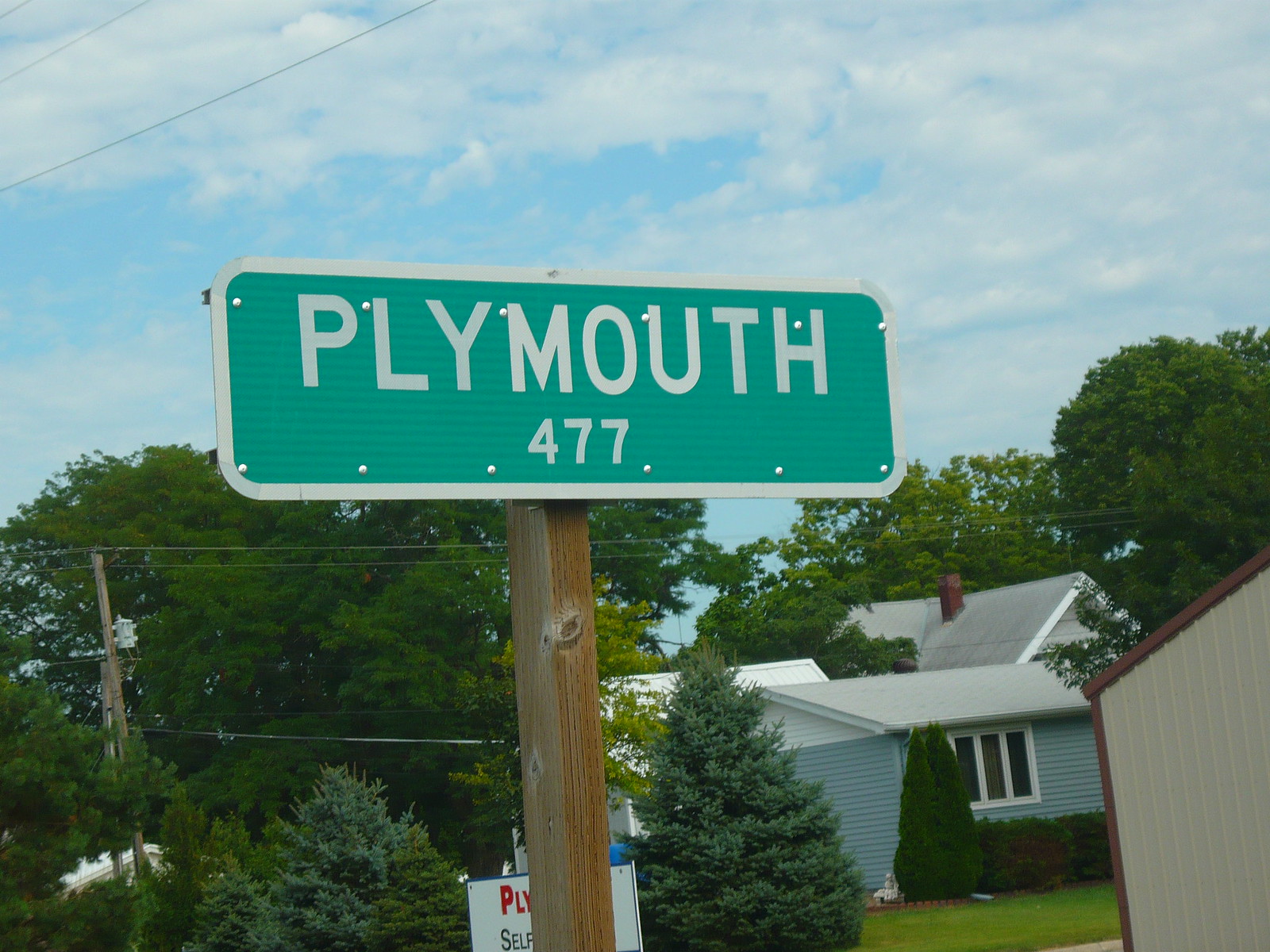In the daytime photograph, a green and white street sign indicating "Plymouth 477" is mounted on a cylindrical wooden pole in a residential area. The sign is designed with white letters on a green background and outlined with a white border on a metal plate. The wooden pole has a somewhat square, cylindrical shape. In the background, a blue and white house with a gray roof can be seen, situated among several mature trees, including pine trees. Partially hidden behind the main sign, there's another white sign with the partial text "PLY" and "SELF." Additional background elements include portions of other buildings and visible power lines that contribute to the residential setting.